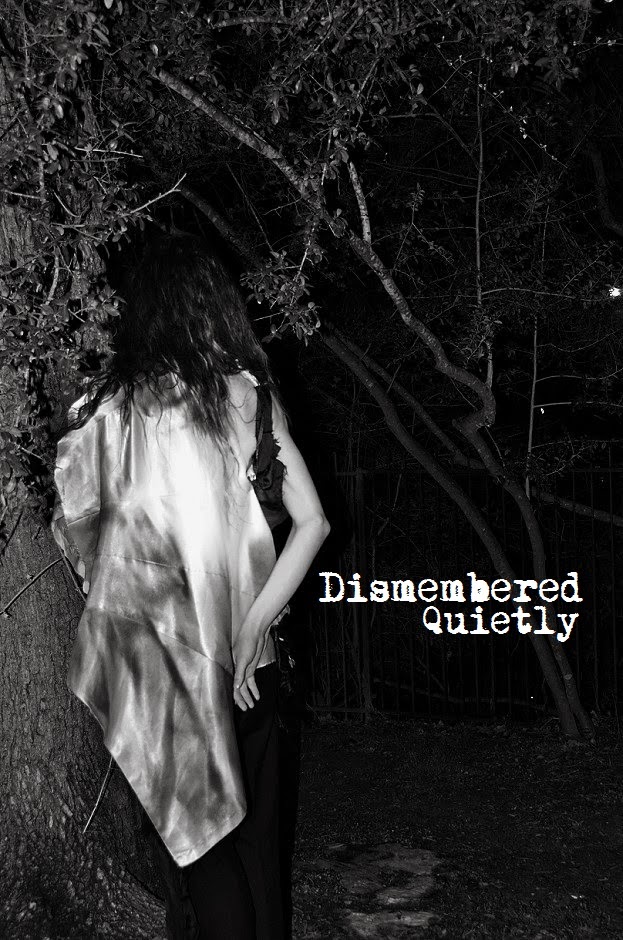In this haunting black-and-white image taken at night, a woman with her back to the camera stands amidst a dark forest. She has long, straight black hair that reaches down past her shoulders, partially covered by a white satin material draped over her left side. She appears to be wearing a black, possibly sleeveless, dress. Her right arm is visible, bent slightly behind her back, resting on the satin material. To her left, a large tree trunk stretches up and across the frame, while thinner trees with small leaves and intertwining branches fill the background on the right. The ground beneath her is dirt, adding to the eerie atmosphere. Over her right arm, two lines of white, grainy-font text read: "dismembered quietly," evoking an ominous mood.